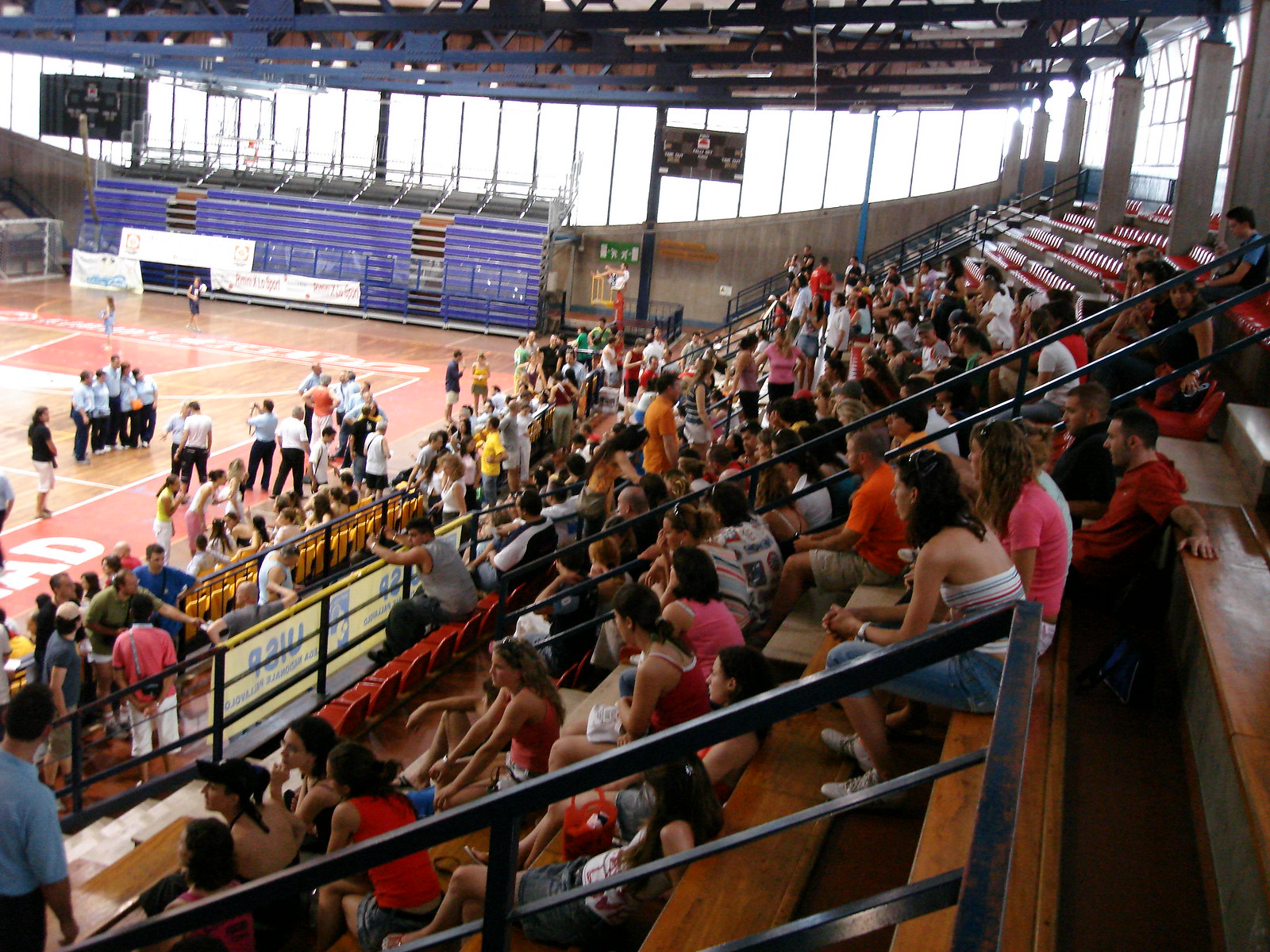The image depicts an indoor athletic event inside a spacious gymnasium or stadium. The photograph is taken from an upper level, providing a comprehensive view of the venue. The primary focus is on a hardwood basketball court with red outlines, which occupies the left side of the image. Several people are standing on the court, likely waiting for a game to start or gathered post-game. 

To the right of the court, rows of spectators are seated on dark brown wooden bleachers with black railings, clad in varied attire of orange, pink, and white shirts. Above these bleachers, in the upper right corner, is a series of large windows supported by white columns, illuminating the arena with natural light. The gymnasium's ceiling features metal rafters painted navy blue.

In the upper left corner, there's a row of blue, retracted temporary bleachers, suggesting additional seating capacity when needed. Below these bleachers, a white archway, possibly made of stone or wood, serves as an entrance for players. A scoreboard is visible near the top, anchoring the scene as participants and spectators prepare for or wrap up an athletic contest.